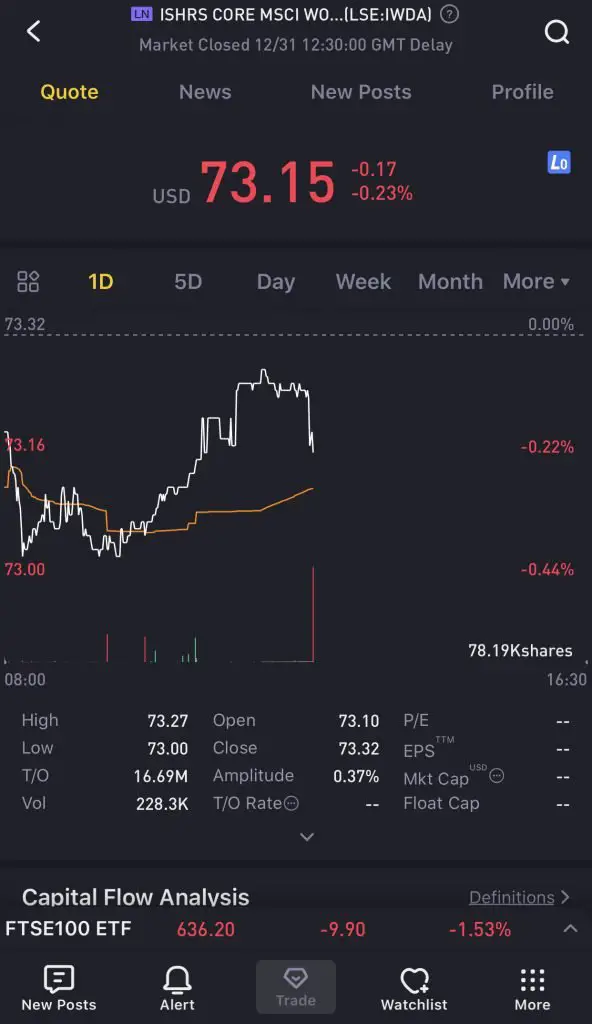Screenshot of a financial app on a smartphone, displaying detailed stock information for ISHR MSCI, listed on the London Stock Exchange (LSE). The screen prominently features a line graph tracking the stock's performance over a one-day period, with options to view data over different timeframes (1D, 5D, Day, Week, Month). The current stock price is USD 73.15, with a decrease of 0.17 points or 0.23%, indicated in red font. 

At the top, the user has navigated to the "Quote" section from the available submenu options, which include Quote, News, New Post, and Profile. Additional details such as "Mark as Closed" are displayed near the top of the interface. 

Below the graph, financial details including the stock's high, low, turnover, volume, open, and close prices are presented. At the bottom of the app, there are further navigation options labeled New Posts, Alert, Trade, Watchlist, and More. The current interface displayed belongs to the "Trade" section, highlighted as the active menu option.